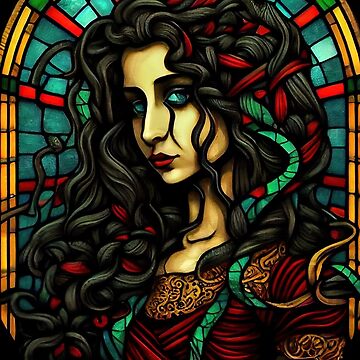This detailed painting depicts a woman positioned against an arched stained glass window. Her dark, wavy hair cascades intricately, interspersed with strands of red and adorned with a green ribbon on the right side. Some of her hair falls over her right eye, partially obscuring one of her striking bright blue eyes. She wears vivid red lipstick, and her head tilts subtly to the left. The woman is dressed in a maroon gown featuring a gold collar with an intricate dark blue design. The ruched fabric of the dress flows elegantly, and two ribbons drape over her chest. Behind her, the arched window features an ornate gold exterior frame, while the interior is composed of aqua-colored squares intersected by red lines.